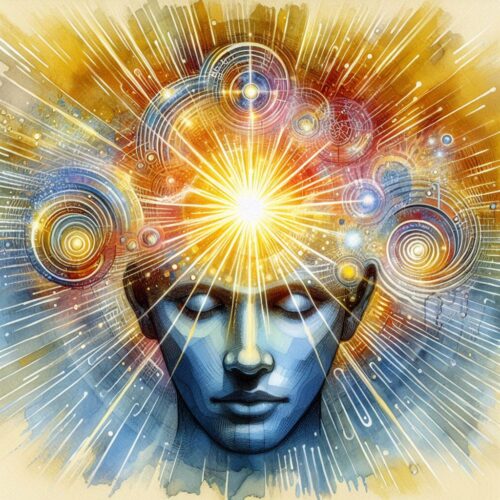This vibrant and mesmerizing image depicts a person's blue-colored face situated slightly below the center, with their eyes closed or looking downward. The focal point is a radiant, sunburst-like design on their forehead, emanating bright yellow rays that form a large circle. Surrounding their head and face are an array of lights, bubbles, and swirling circles in hues of yellow, blue, orange, and purple, giving the impression of cosmic or mind-expanding energy. The composition extends outward, with rays of light radiating in all directions at the top and bottom of the image, contributing to the trippy, almost otherworldly atmosphere that evokes a sense of a merging galaxy and a profound, contemplative state.